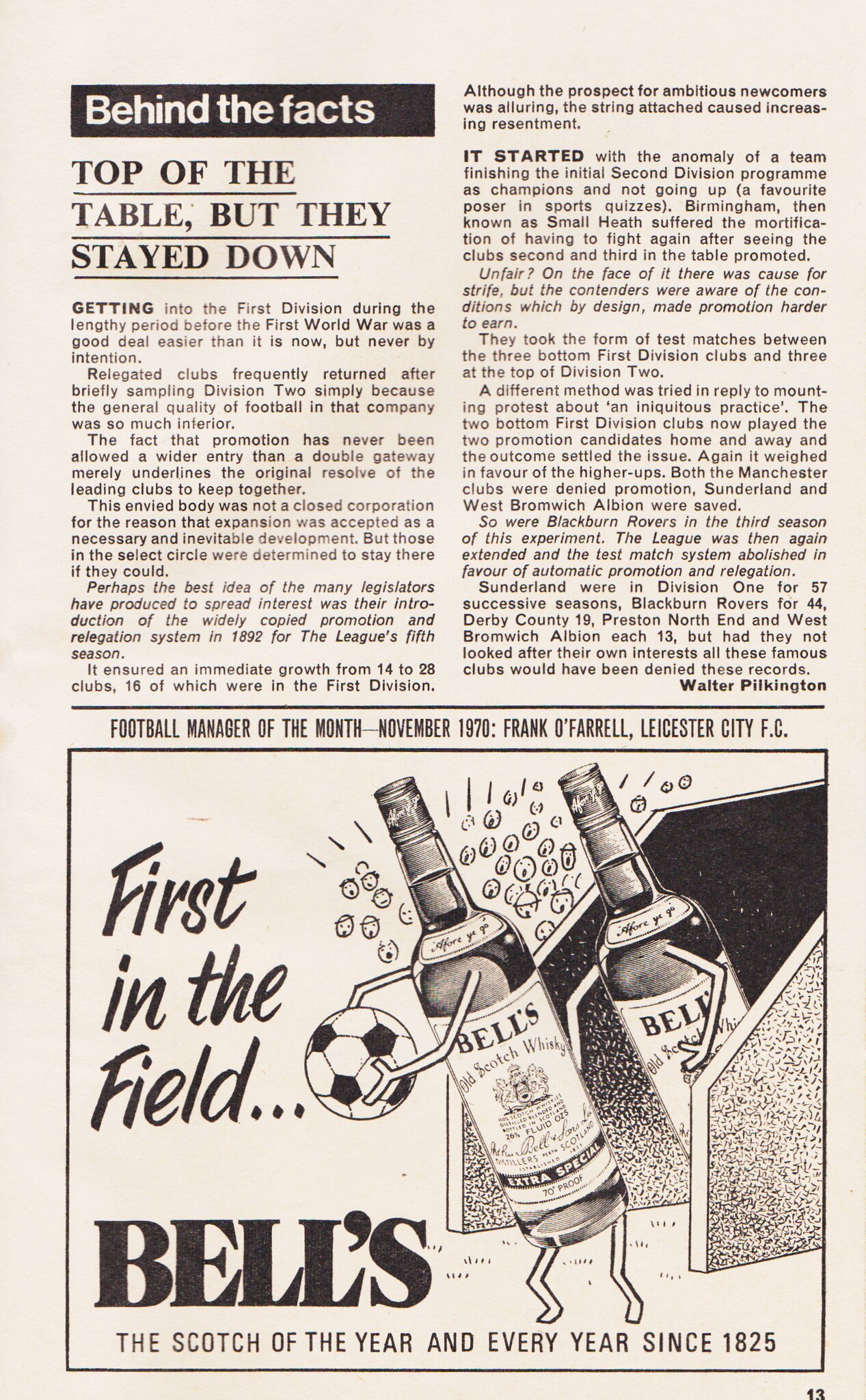This detailed image appears to be a tall rectangular excerpt from a newspaper or a poster, featuring distinct sections of text and an advertisement. The background color is a light beige. At the top of the image, there are two columns of text. The left column begins with a black rectangle containing white font that reads "Behind the Facts." Beneath that, in large, bold, all-capital black letters, it reads "TOP OF THE TABLE, BUT THEY STAYED DOWN." This header is followed by several paragraphs of small black text, spanning two columns.

Below this main text, another bold, all-capital title reads "FOOTBALL MANAGER OF THE MONTH, NOVEMBER 1970, FRANK O'FARRELL, LEICESTER CITY, F.C." Underneath this title, an advertisement is framed by a black rectangle. The ad features an illustration of two bottles of whiskey entering a soccer field, with one bottle holding a soccer ball. The text within the ad reads "First in the Field... Bell's Old Scotch Whiskey, Extra Special." Additionally, it mentions "Bell's Scotch of the Year—and Every Year Since 1825." The advertisement also depicts the faint faces of a cheering crowd in the background.

The consistent black, white, and shades of gray color scheme, coupled with the detailed historic and promotional content, gives the impression that this image was sourced from an old magazine, newspaper, or perhaps a vintage informational poster.